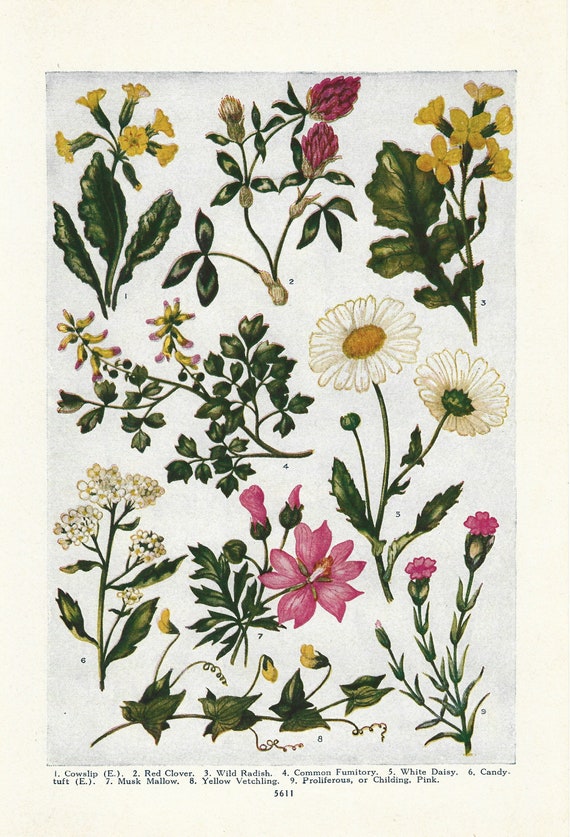The image depicts a vintage botanical illustration, presented as a flower identification poster. Enclosed in a thick white frame, the poster features a light blue background, with colorful illustrations of various wildflowers. Each of the ten flowers is numbered and identified with its name at the bottom of the poster. Notable flowers include cowslip, red clover, wild radish, white daisies, yellow vetchling, and what look like marshmallow, yellow tubular flowers, pink phlox-like flowers, and dainty white florets. The overall palette consists of muted hues of pink, yellow, green, and white, lending the illustration a soft, vintage aesthetic. The detail and key at the bottom emphasize its purpose for flower identification, indicating its use as an educational or decorative piece.